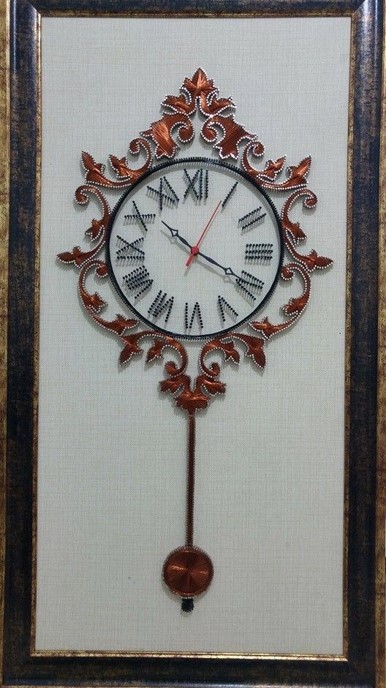This striking photograph, oriented in a portrait view, captures a close-up of a framed picture of a vintage clock. The frame is rectangular, adorned with a sleek black finish, accented by a rich copper-colored border. At the center of the framed picture is a black circular clock face, featuring elegant black Roman numerals. A prominent copper-colored line extends down from the clock, culminating in a rounded ornament beneath it. Surrounding the clock is an intricate, copper-colored ornate design, adding to the antique charm. The entire composition is set against a serene light gray background, highlighting the details and contrast of the frame and the clock.